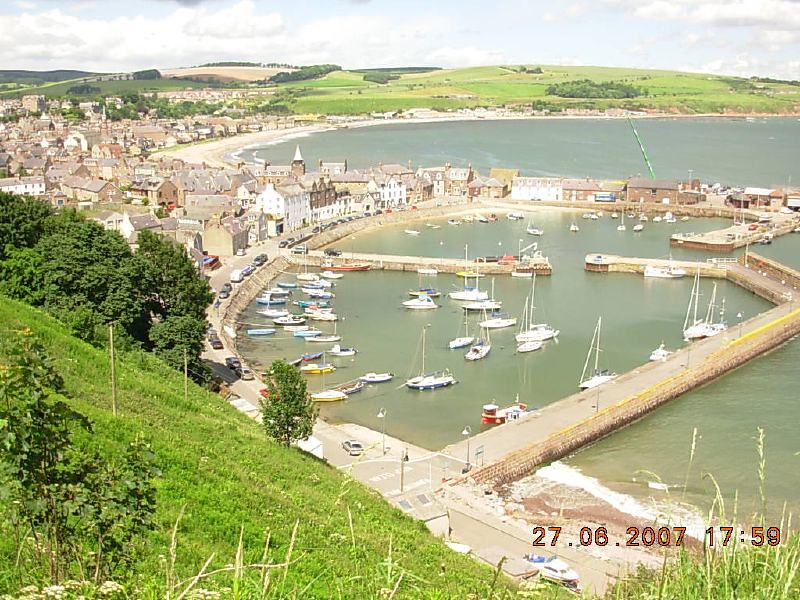This is a detailed aerial view of a marina at the seaside, captured in a color photograph dated June 27, 2007, at 5:59 PM. The image, taken from a drone in landscape orientation, shows a pie-shaped marina with numerous boats, some with sails, moored in the water. The marina is connected to an adjacent body of water, surrounded by a wall, with passageways leading to the open ocean. In the foreground, a street lined with cars curves around the shoreline, and near the bottom left, there's a green grassy slope. Towards the top left, a village with multiple houses and rooftops is visible. The horizon features expansive green hillsides, adding to the lush vegetation that surrounds the landmass areas visible in the photograph. The various elements of the image harmonize to form a picturesque seaport scene with a rich blend of natural and man-made structures.